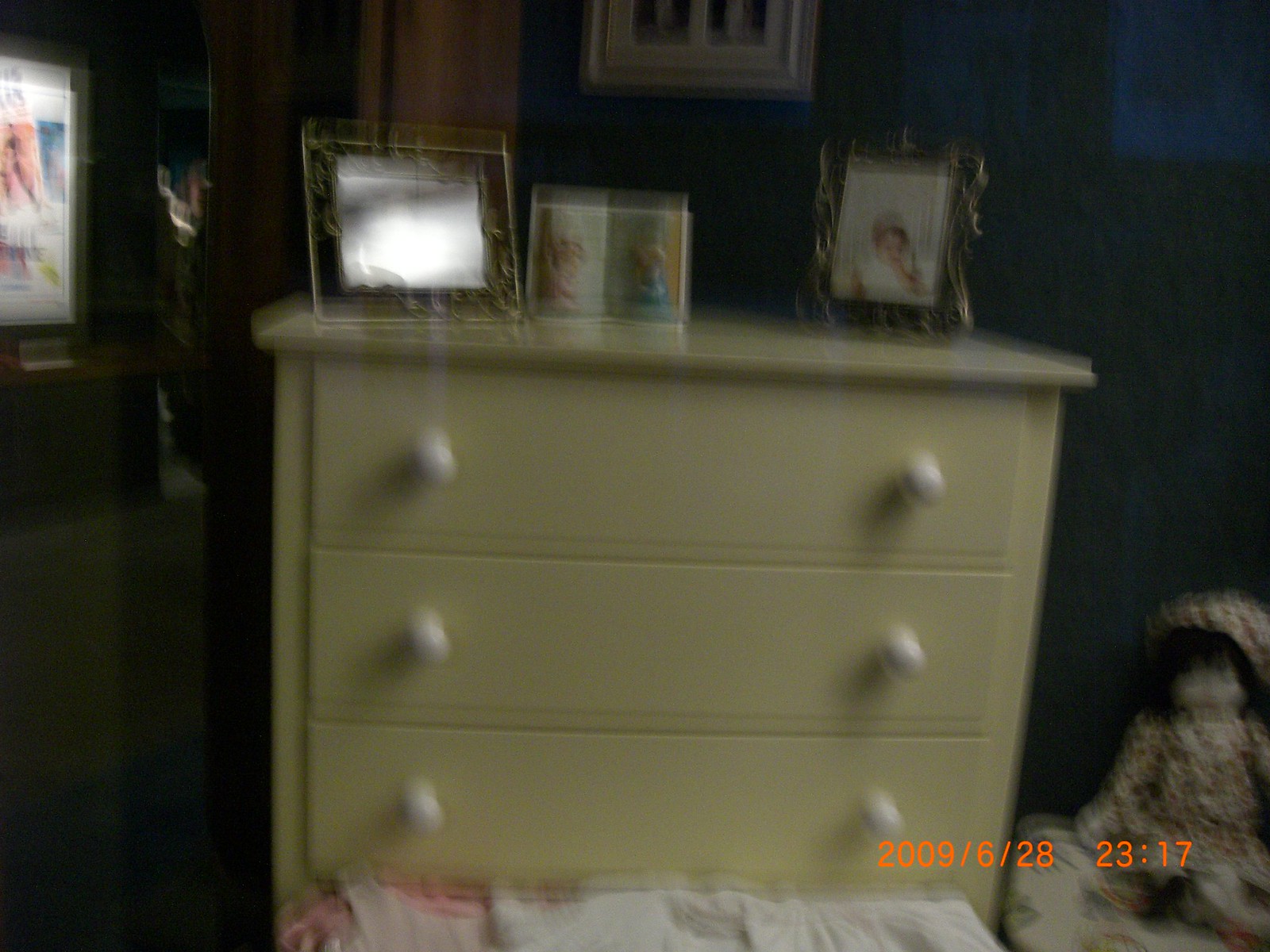The image captures a dimly-lit room featuring a light tan dresser with three visible drawers, each adorned with two white knobs. Atop the dresser, there are three framed pictures arranged neatly. To the left edge of the dresser stands a trophy, which gleams subtly, hinting at a possible achievement. In the bottom right corner of the image, a doll is delicately seated on a small chair. The timestamp at the bottom of the image indicates it was taken on June 28, 2009, at 23:17. In the background, the wall is adorned with various pictures, though they are not clearly discernible due to the overall blurriness of the photograph.